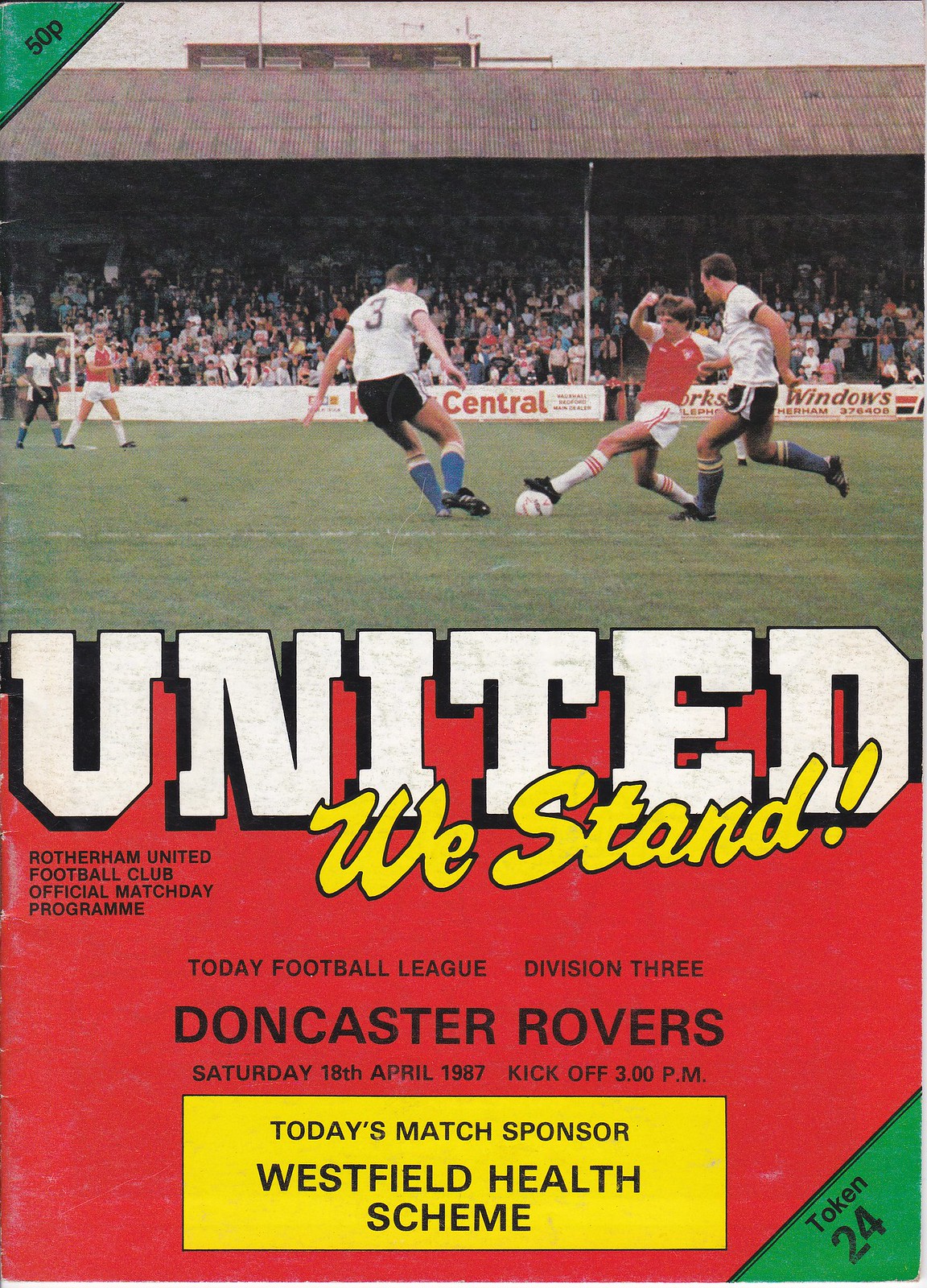The image is a scanned cover of an official match day program from an old soccer game, featuring the Rutherham United Football Club. In the foreground, a player in a red uniform with black sneakers and white socks, featuring red bands, is captured in the midst of kicking a soccer ball. He is closely pursued by players from the opposing team, who are wearing white tops and black shorts. The scene takes place on a grass field, with a full stadium of spectators in the background. The audience is partially obscured by signs that read "Central" and "Windows," barely visible behind the action.

Below the image of the game, the text "United We Stand" is prominently displayed against a red background. Underneath, it reads in smaller black text: "Rutherham United Football Club official match day program." Further details include "Football League, Division 3, Doncaster Rovers," along with the date "Saturday, 18th April 1987," and the kickoff time "3 p.m." A yellow rectangle beneath this information announces "Today's match sponsor: Westfield Health Scheme." In the bottom right corner, a green triangle designates "Token 24," and a "50p" price appears in the top left corner.